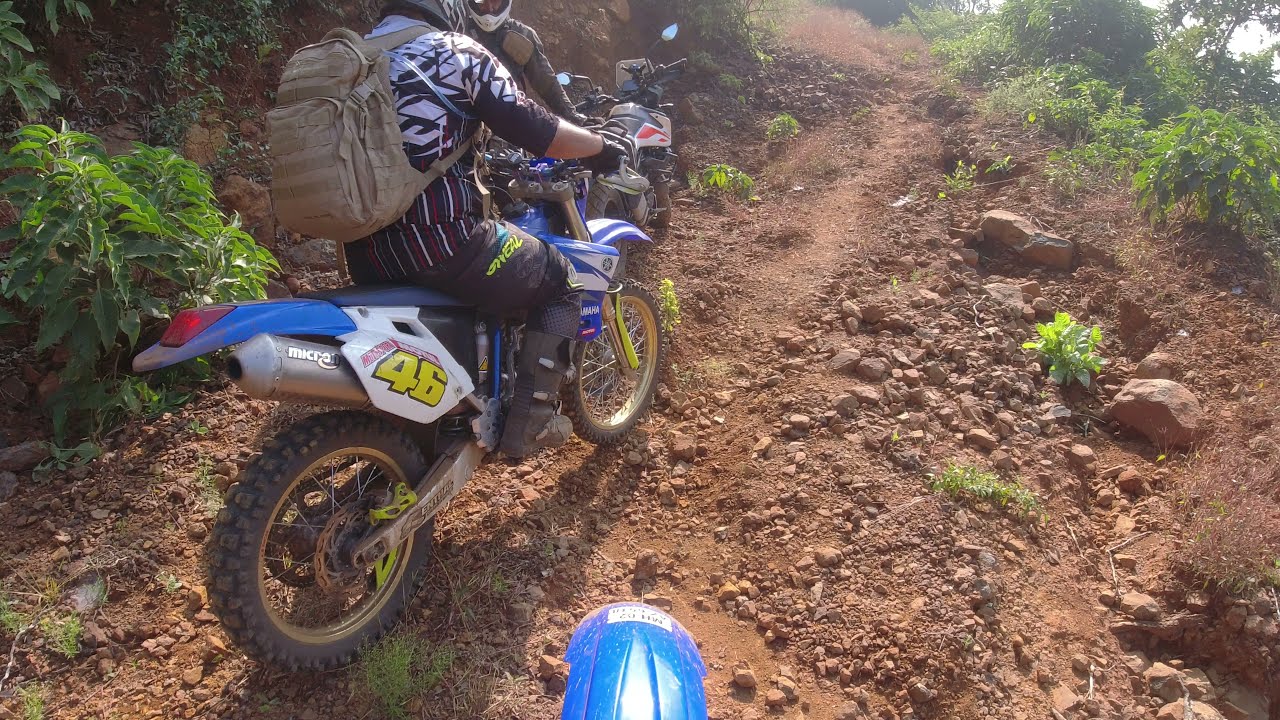On a narrow, rugged dirt trail lined with gravel and rocks, you find yourself riding a dirt bike, evidenced by the blue fender visible at the bottom center of the frame. The trail is flanked by greenery, including bushes and trees, creating a natural, immersive setting. Ahead and slightly to the left, another dirt biker is riding a blue and white motorcycle marked with the yellow number 46. This rider is clad in dark pants, long dark boots, and a three-quarter length white and black striped shirt, along with a beige/brown backpack. In front of him, another rider has parked his dirt bike and stands facing the first biker. This second rider is partially obscured, but can be identified by his white helmet and dark shirt. Beyond them, the dirt trail continues into the distance, bordered by a mix of green grass and trees. The perspective suggests the image was captured from a helmet-mounted camera, offering a dynamic view of the dirt biking adventure and the surrounding natural landscape.